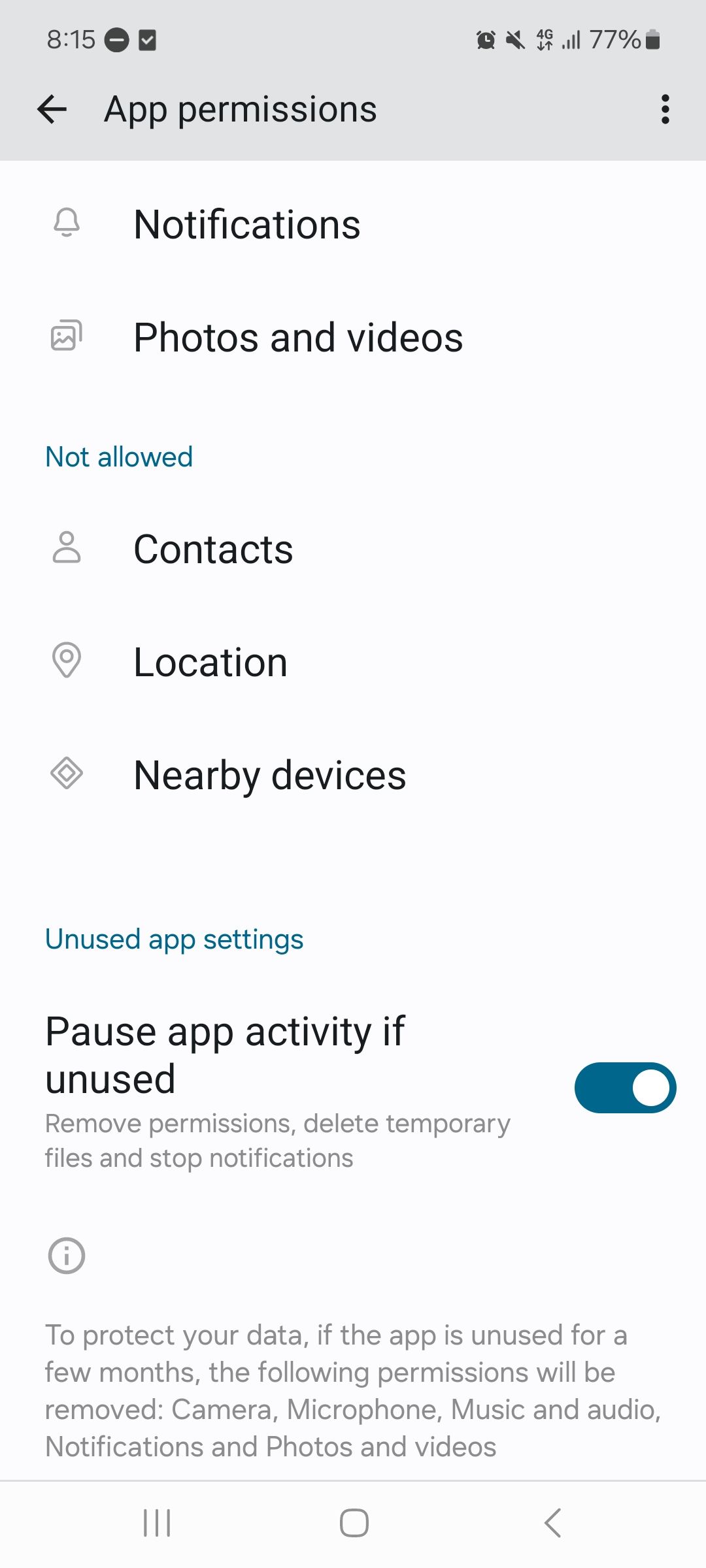This is a vertical rectangular image, apparently a screenshot taken from a cell phone. It has a narrow aspect ratio typical of mobile screens. At the top, there is a gray rectangular status bar displaying the current time "8:15" on the left, and various status icons, including a battery icon indicating 77% charge, on the upper right corner.

Just below this status bar, aligned slightly to the right from the left edge, the header text reads "App Permissions" with a right-pointing arrow next to it. On the far right side of this header, there are three vertical dots indicating additional options.

The main content of the image is set against a white background and lists various app permissions. Below the "App Permissions" header, there is a series of permissions, each associated with a little icon to the left and descriptive text in bold black font to the right. These permissions start with "Notifications" followed by "Photos and videos," both of which have the status "Not allowed" displayed in a teal font, left-justified under the permissions.

Next, listed in bold black font are "Contacts," "Location," and "Nearby devices," with no accompanying status indications. Further down, another teal-colored section reads "Unused app settings," and below it, in black font, "Pause app activity if unused" is specified.

Underneath this, small gray text explains the effects of pausing app activity: "Remove permissions, delete temporary files, and stop notifications." To the right of this explanation is an on/off toggle switch, which is set to 'on,' as indicated by a white circle pushed to the right and the teal-colored section exposed to the left.

Lower down, there is a small gray circle with an eye icon inside, set against a white background. Finally, light gray text provides additional details: "To protect your data, if the app is unused for a few months, the following permissions will be removed: camera, microphone, music and audio, notifications, and photos and videos."